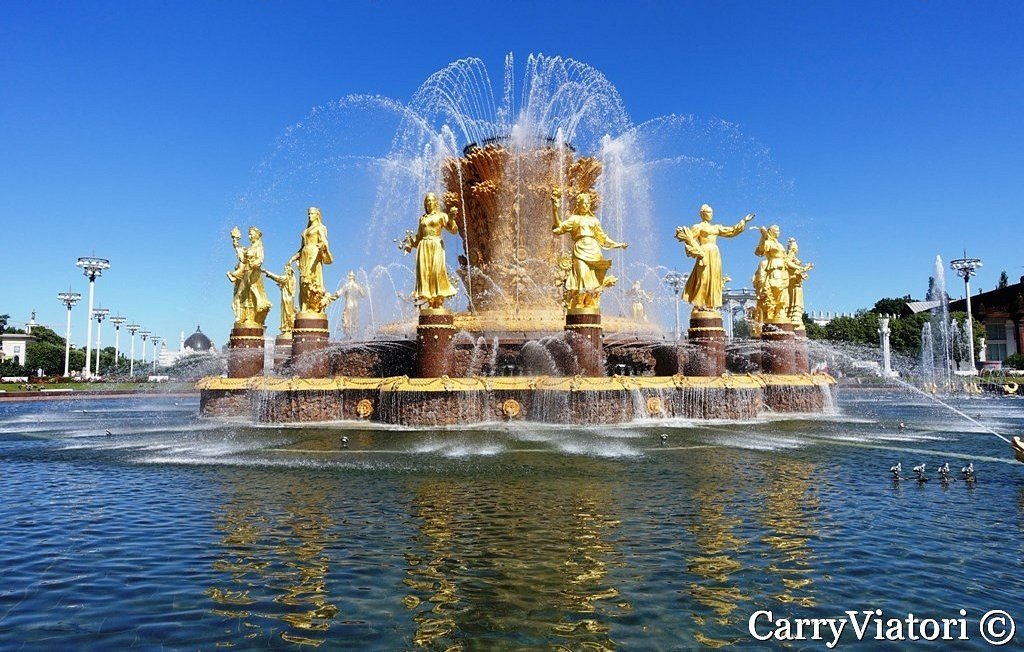The image captures a grand, circular fountain surrounded by a tranquil pond with ripples, reflecting a vibrant blue sky. Nine gold-colored statues, each positioned on individual stands, encircle the fountain. Water elegantly sprouts from the top, sides, and base of the fountain, creating a mesmerizing spray. The fountain structure features a brown and yellow palette, with a notable yellow strip around its base. In the background, a row of large white structures, possibly stadium lights, are faintly visible. Also present in the scene are a few ducks gliding on the water. The bottom right-hand corner of the image bears the white text "Cary Viatori," indicating a copyright marking. Possibly set in a European locale, the ambiance is enhanced by the pristine weather, adding to the fountain’s splendid appearance.